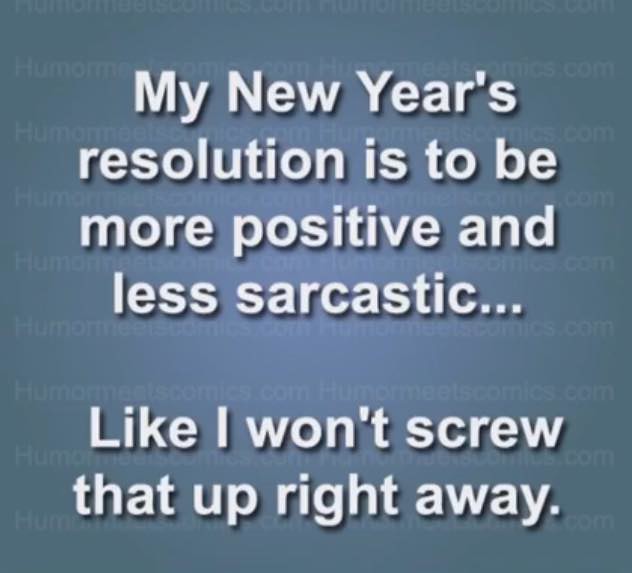The image features a light blue-gray background with a humorous New Year's resolution. The resolution states, "My New Year's resolution is to be more positive and less sarcastic. Like I won't screw that up right away." This text is presented in white letters with a subtle black shadow, arranged in two blocks: the first block consists of four lines at the top, and the second block has two lines at the bottom. Throughout the background, there is a barely noticeable, ghosted-out text repeating "Humorlesscomics.com." The overall appearance suggests this could be a snippet from a social media post or a webpage, designed with a clean, modern aesthetic.